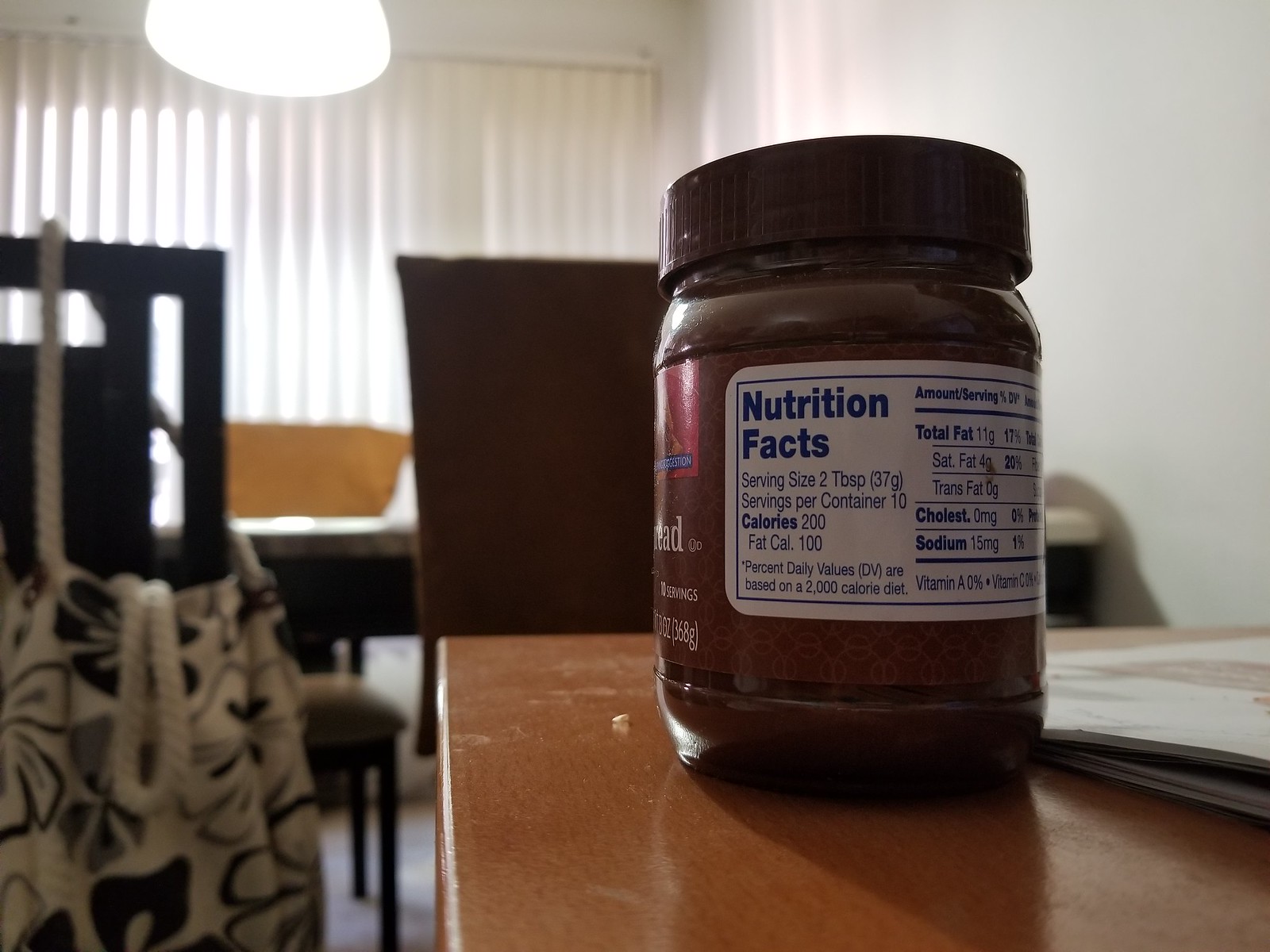In this color photograph taken indoors, a polished brown wooden table dominates the foreground. Placed on the table is a bottle with its back facing the camera, revealing a white label with blue text detailing the nutrition facts. The brown bottle, featuring a matching brown lid, lists its contents in servings of 2 tablespoons, with 10 servings per container, 200 calories, and 100 calories from fat.

Beyond the bottle, vertical drapes run along the background, adding a sense of depth to the scene. In front of the table, a chair holds a white and black striped satchel, casually hung over its back. Additional chairs are visible in the distance, suggesting a communal or dining area. Scattered on the table are some pieces of paperwork, adding an element of everyday activity to the setting.